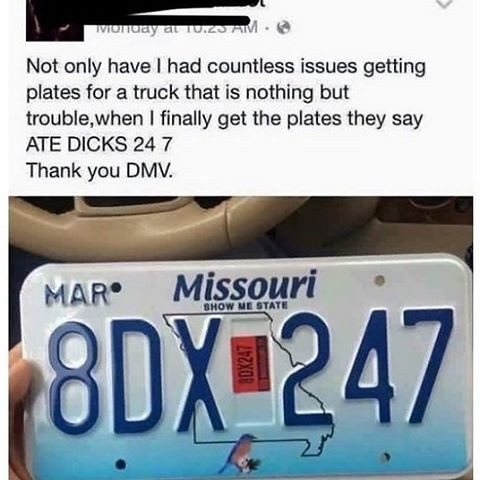The image is a screenshot of a social media post venting frustrations about obtaining license plates for a troublesome truck. The post, with the author's name blacked out, reads: "Not only have I had countless issues getting plates for a truck that is nothing but trouble, when I finally get the plates, they say 8 dicks 24 7. Thank you DMV." Below this text, there's a photograph showing a hand holding a white Missouri license plate with blue text that reads "8DX247". At the top of the plate, "Missouri" is printed in blue, along with "Show-Me State". There are various details including an outline of the state of Missouri, an orange sticker indicating the month of March in the left-hand corner, a state bird image, and the bottom edge of a beige steering wheel in the top left corner of the photo.